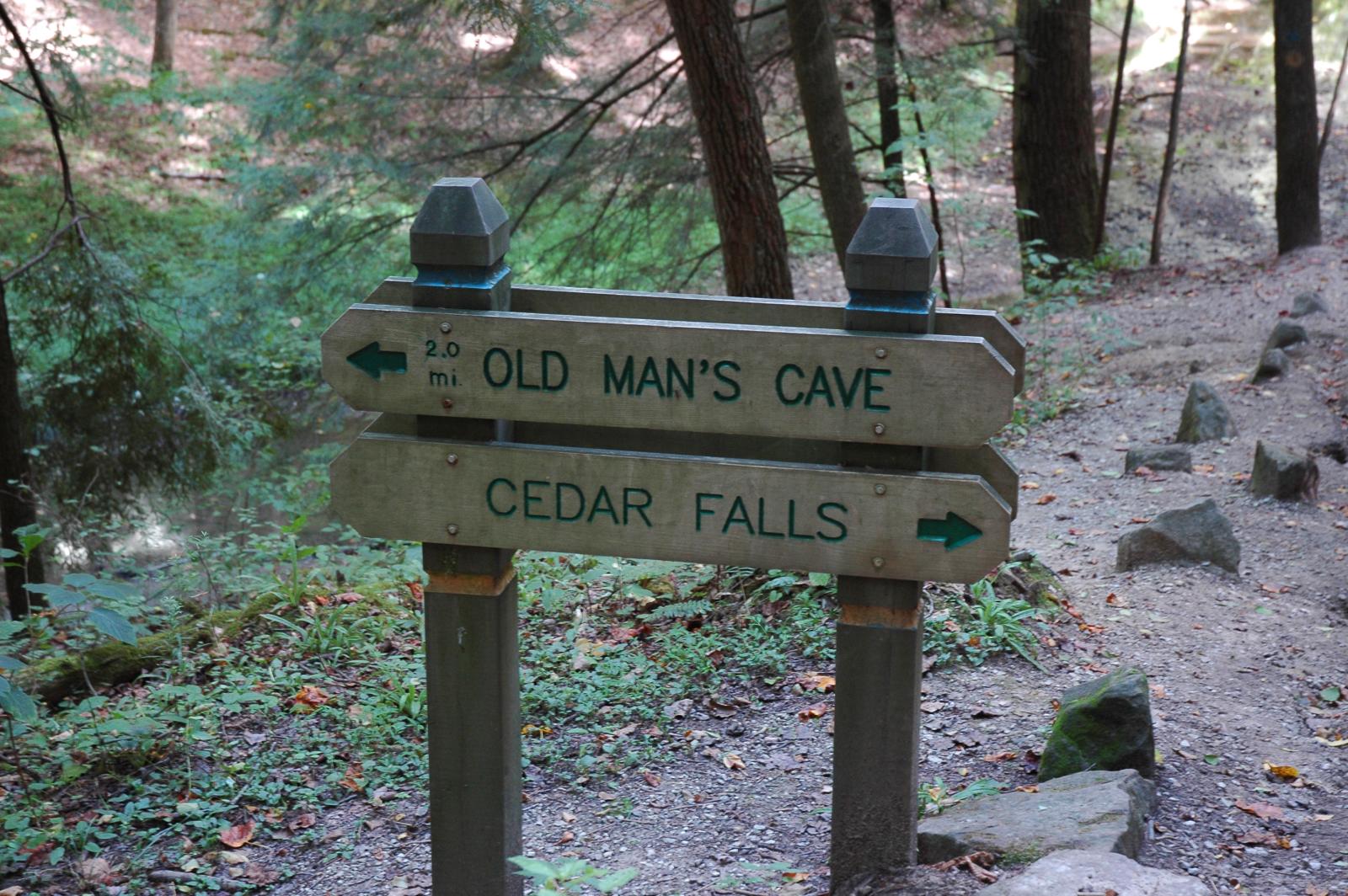This photograph captures a serene forest environment, emphasizing a central wooden signpost with metal plaques. The signpost stands on a woodland path, surrounded by towering pine trees, lush green foliage, a meandering stream, and scattered rocks. The text on the sign indicates directions to Old Man's Cave, 2.0 miles to the left, and Cedar Falls to the right, with both destinations marked by arrows. The sign itself is brown with green text, enhancing its natural integration with the surrounding scenery. This picturesque moment, likely taken by a hiker enjoying the tranquility and beauty of the forest trail, highlights the natural hues and textures, creating a vivid and detailed portrayal of the hiking experience near Old Man's Cave and Cedar Falls.